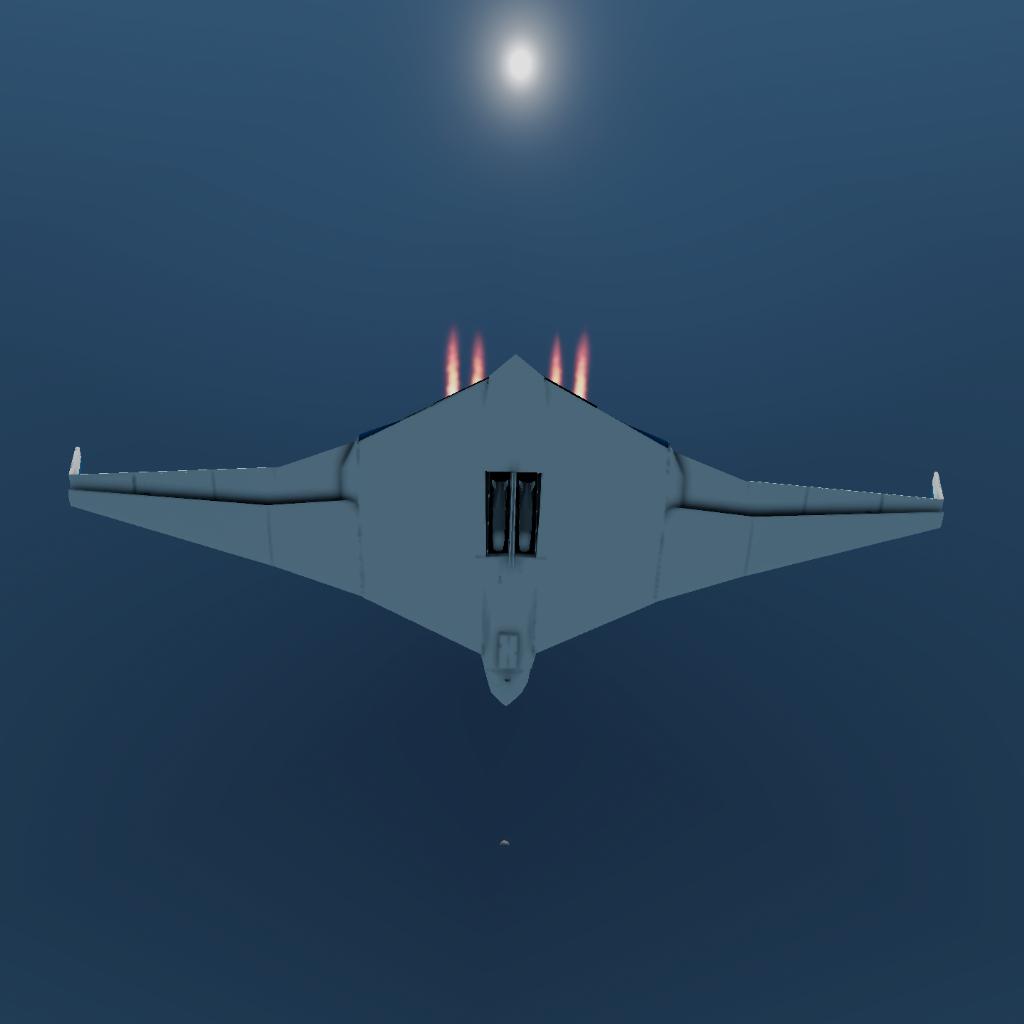The image depicts a computer-generated plane, resembling a B-2 bomber or spy plane, flying through a dark blue sky. The aircraft has a flying wing design with a light blue, almost diamond-shaped body and large, slightly triangular wings extending from either side. The plane's nose is oriented towards the bottom of the image, while the tail end points upward. At the rear, there are four orange and yellow jet flames emanating from the engines. In the center of the aircraft, two black vertical lines can be seen, possibly indicating bomb bays or other features. Above the plane, a small, bright white orb, likely the sun or moon, is surrounded by a soft glow, adding a striking contrast to the scene.